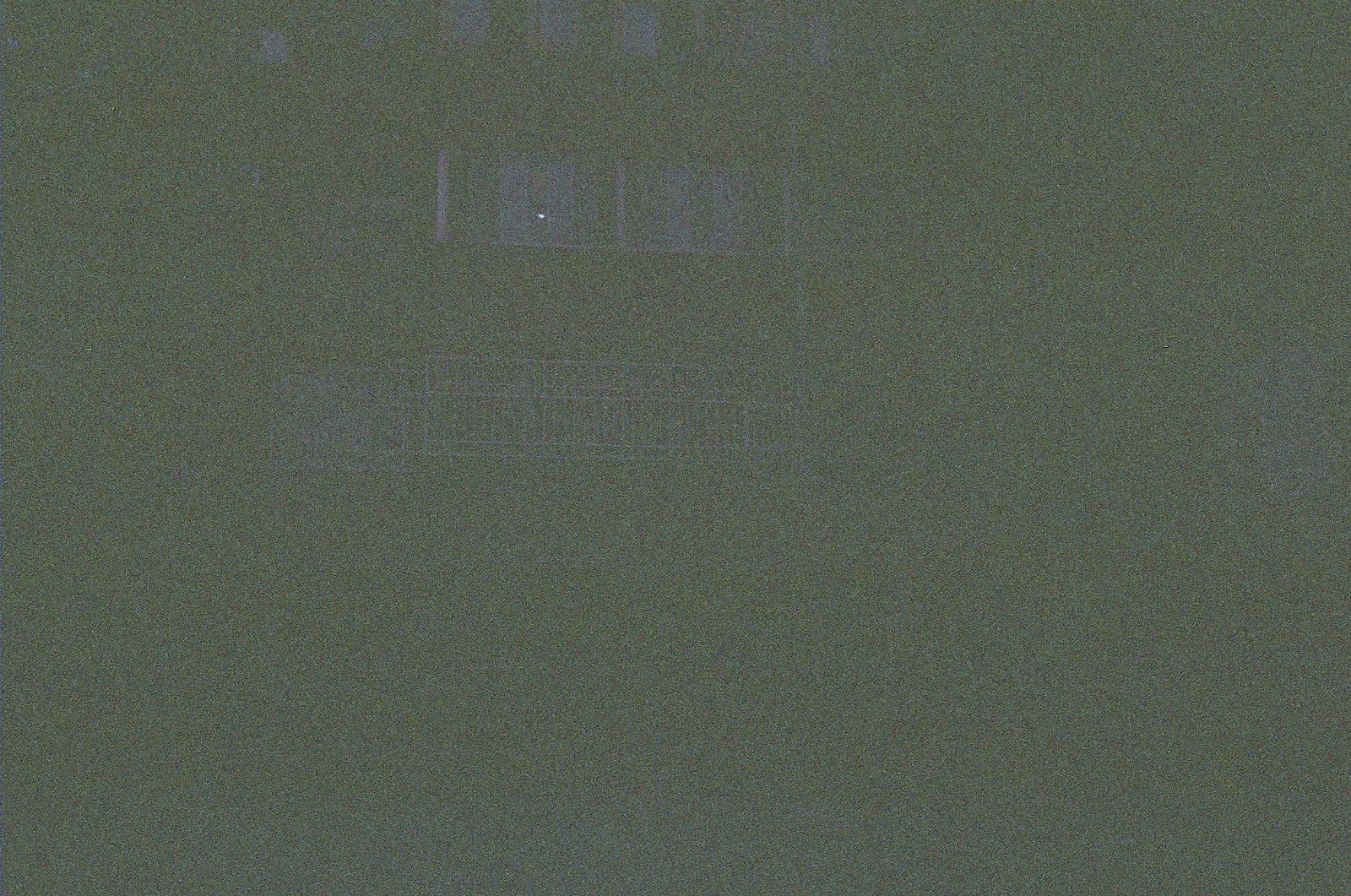This photograph exhibits an extremely grainy texture, reminiscent of static on an old television screen. The image captures the exterior of a multi-level building, shrouded in shades of gray and white, suggesting a snowy environment. A white railing, likely part of a balcony, is faintly visible amidst the graininess. Above the balcony, several windows can be discerned, one of which appears to reflect a flash of white light. The overall aesthetic of the photograph gives an impression of nostalgia and obscured clarity, as though viewed through a vintage lens.